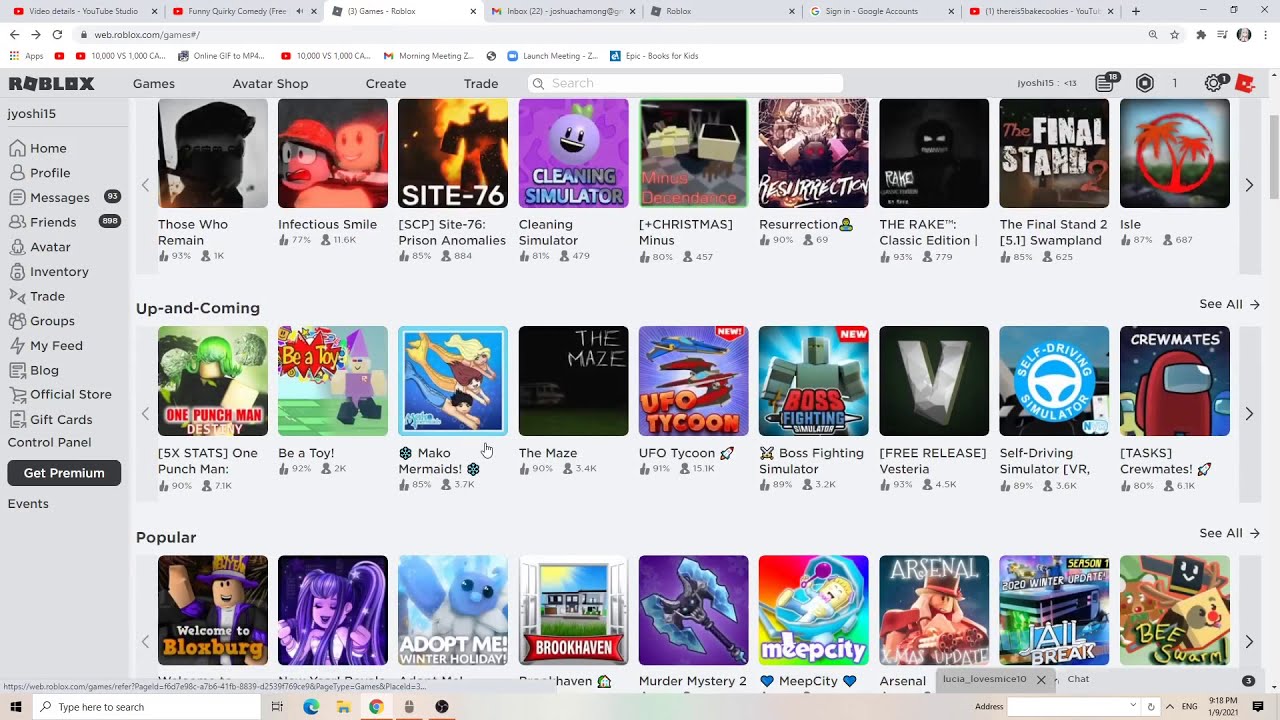The screenshot showcases a dense, right-hand side view of a Roblox interface, filled with multiple open windows and tabs. Numerous categories and options are visibly arrayed, including "Games," "Avatar Shop," "Create," "Trade," and listings for "Up and Coming" and "Popular" games. The user's homepage displays various sections: Home, Profile, Messages (93), Friends (nearly 1,000), Avatar, Inventory, Trade, Group, My Feed, Blog, Official Store, Gift Cards, Control Panel, Get Premium, and Events. Approximately 40 games are displayed in full color, each showing the game's title, the number of likes and plays, spanning genres like robot games, UFO games, and anime games. Below these are icons indicating where each game is playable, with a search bar positioned underneath, all within a Windows operating system environment.